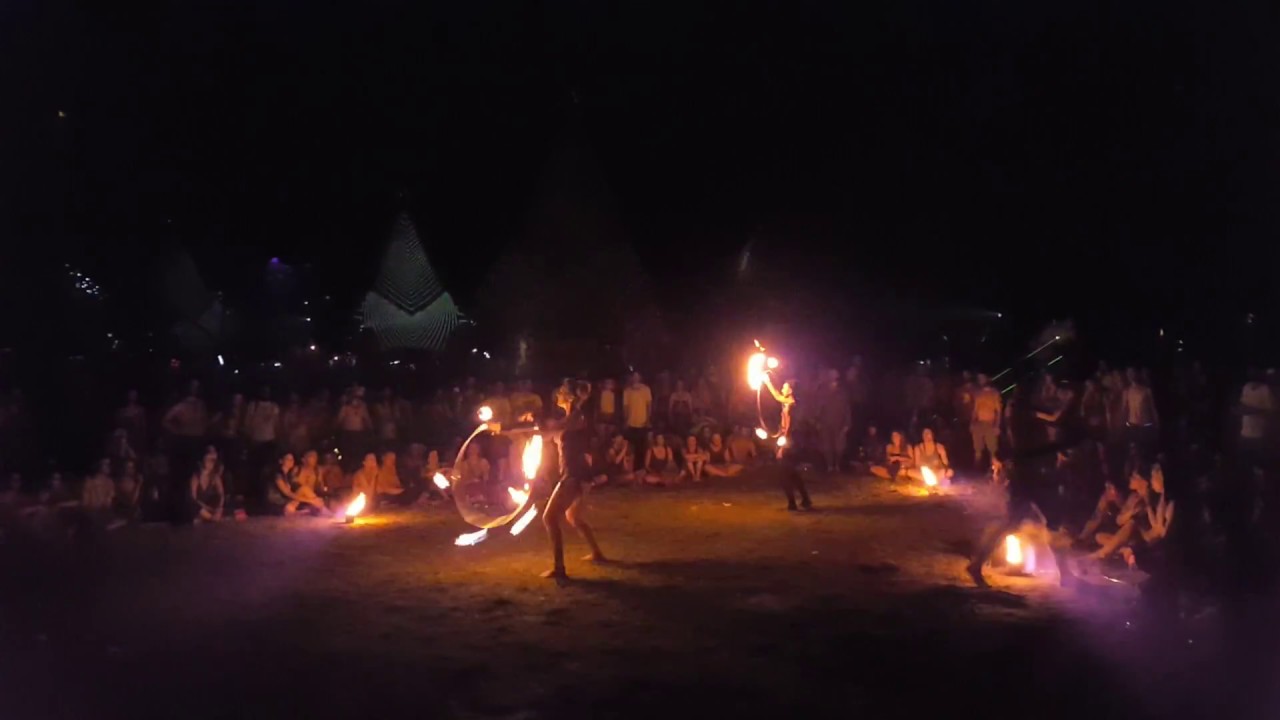This nighttime photograph captures a captivating outdoor event, likely a powwow or ceremonial gathering, highlighted by three intriguing performers engaged in a fire act. Against a backdrop of traditional Native American teepees, which give the scene an authentic cultural ambiance, the performers command attention as they twirl hula hoops lit with blazing fire, creating mesmerizing arcs of light against the pitch-dark surroundings. The audience, consisting of both adults and children, appears to be seated on the ground or standing behind the first row, deeply engrossed in the performance. Despite the image's darkness rendering specific details and individual identities indistinct, the scene is brought to life by the bright, dangerous stunts of the dancers. The presence of perhaps around a hundred spectators, bathed in the fiery glow, adds to the enchanting and somewhat mysterious atmosphere of the event.